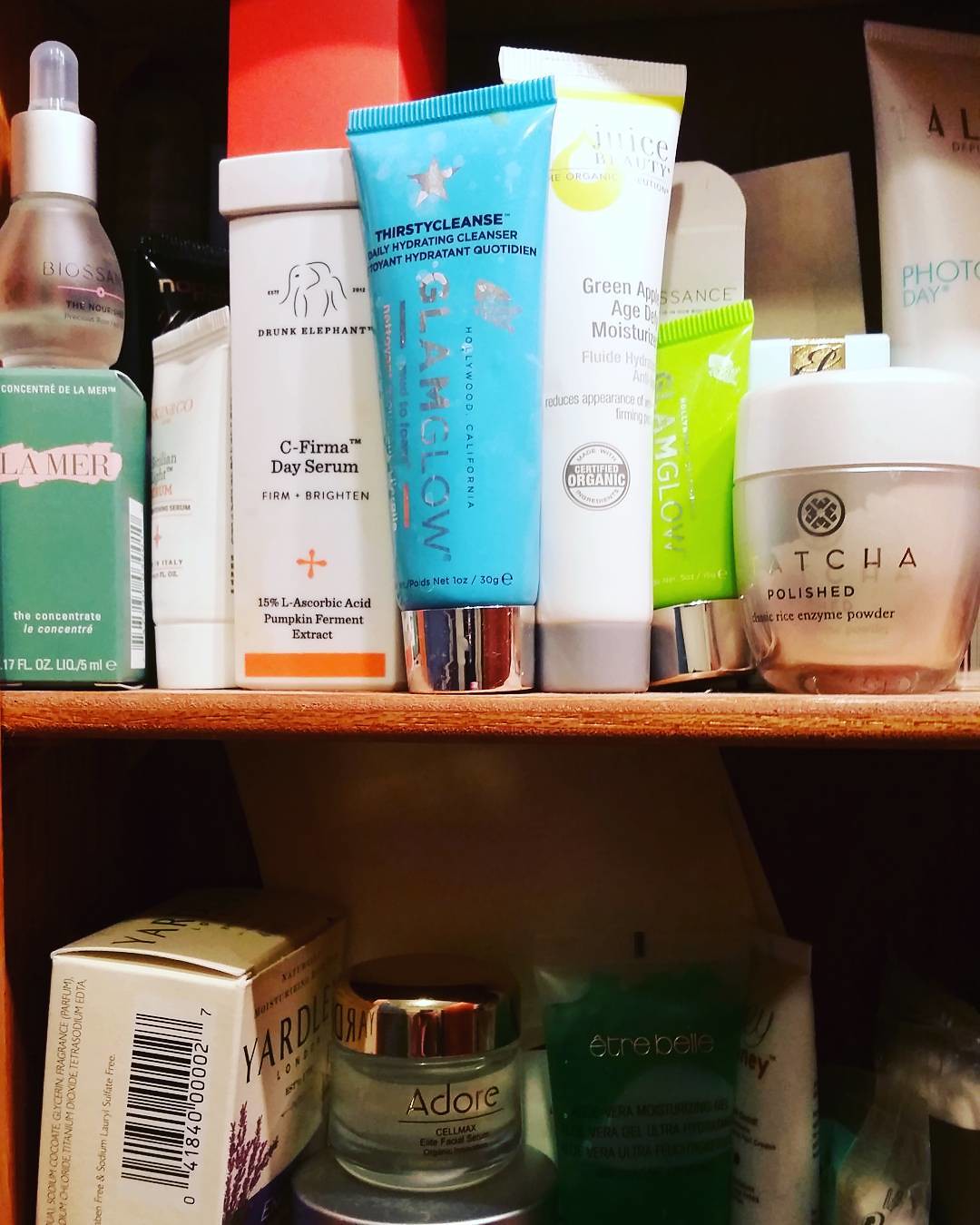This photograph showcases a close-up view of a two-tiered wooden shelf, likely located in someone's home rather than a store, based on the eclectic arrangement of items. The shelf, made of rich brown wood, is filled with an array of personal care products. On the top shelf, the assortment includes white bottles, jars, blue containers, and bottles with green accents, featuring various brands of face lotions, moisturizers, and other skincare items. The bottom shelf houses a boxed bar of Yardley soap on the left, identifiable by its white box adorned with black and purple designs. Additionally, there are several small jars and containers of skin and face creams placed alongside, with a variety of other products visible behind them, partially obscured by those in the foreground. The diverse collection of items, mixed brands, and personal arrangement suggest this is a privately owned shelf, adding a sense of personal touch and daily routine.